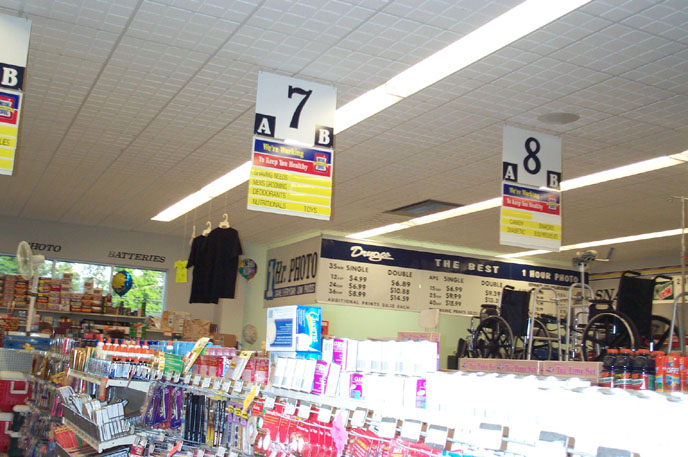The photograph appears to be taken inside a drug store from approximately 30 years ago, specifically showcasing the pharmacy department. On the right-hand side of the image, a white shadow partially obscures some items. In the background, a sign reads "One Hour Photo," while another black label prominently displays the word "Drugs." Black t-shirts hang from the ceiling. The presence of wheelchairs and canes displayed near the ceiling suggests this section is indeed the pharmacy. A white fan is visible, and various medications, including aspirins, are displayed on the shelves. Signs above the aisles indicate their numbers, with aisle 7 and aisle 8 clearly marked. Additionally, assorted razors are also visible in the image.